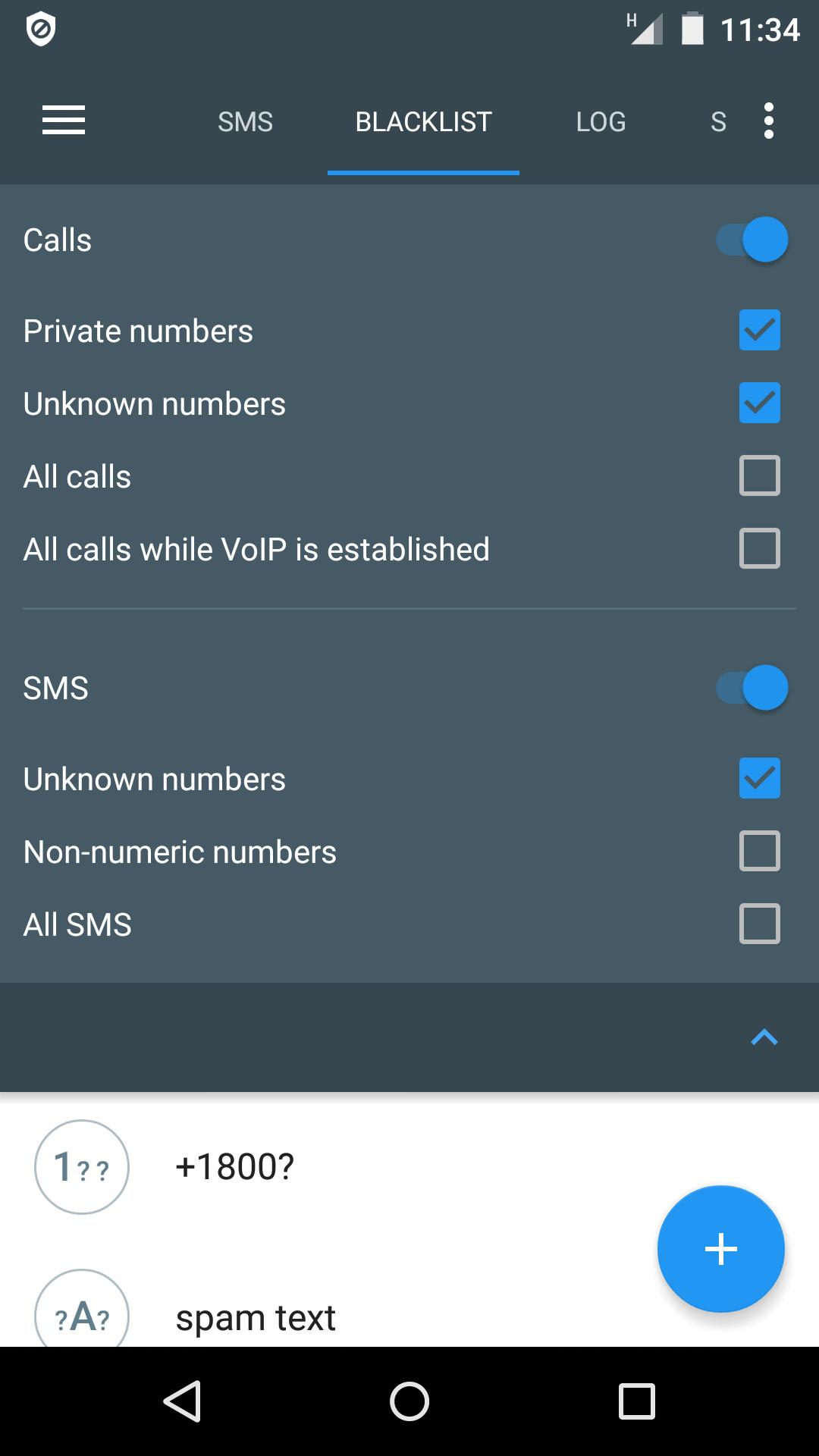In the top left corner of the image, there is an icon labeled "shield." Adjacent to it in the top right corner, an icon labeled "H" appears. The screen displays partial signal strength but a full battery, with the time indicated as 11:34. Several icons and labels are arrayed below, including "SMS," "blacklist," "log," "S," "calls," and "toggle." 

The image highlights settings for private numbers with a blue checkmark next to them, and unknown numbers also have a checkmark. However, "all calls" and "all calls with your IP established" are not checked. The "SMS" option is toggled on, with unknown numbers checked and non-American numbers unchecked. The "all SMS" option remains unchecked.

There is a message with multiple question marks, including "+1803?" and a sequence of question marks that appear as placeholders or unrecognizable input. A spam text indication is marked with a blue circle containing a plus sign.

At the bottom of the screen, a black bar extends across with several interface elements, including an arrowhead triangle pointing left, a circle, and a square, followed by the text "vis-a-vis." The bar and surrounding elements are shaded in gray. Near the bottom, "vis-a-vis smartphone" and menu items are partially visible.